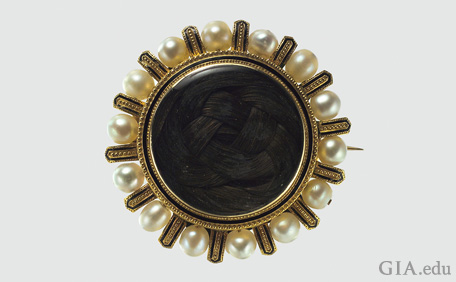This photograph captures an intricate, antique brooch set against a cream and mint-green background. The brooch is prominently circular, featuring a central black stone that is possibly onyx, ensconced within a gold or bronze metal border. The black stone has a cloudy, swirly appearance with faint interwoven patterns. Radiating from this center are gold or bronze tabs or spikes, each bordered with black enamel paint and alternating with luminous, creamy white pearls. This alternating pattern of metal tabs and pearls creates a striking sunburst effect around the brooch. On the right side of the image, a thin, sharp clasp, indicative of a brooch, peeks out discreetly. In the bottom right corner of the photo, the text "GIA.edu" is visible in gray capital letters, adding an educational touch to the image.